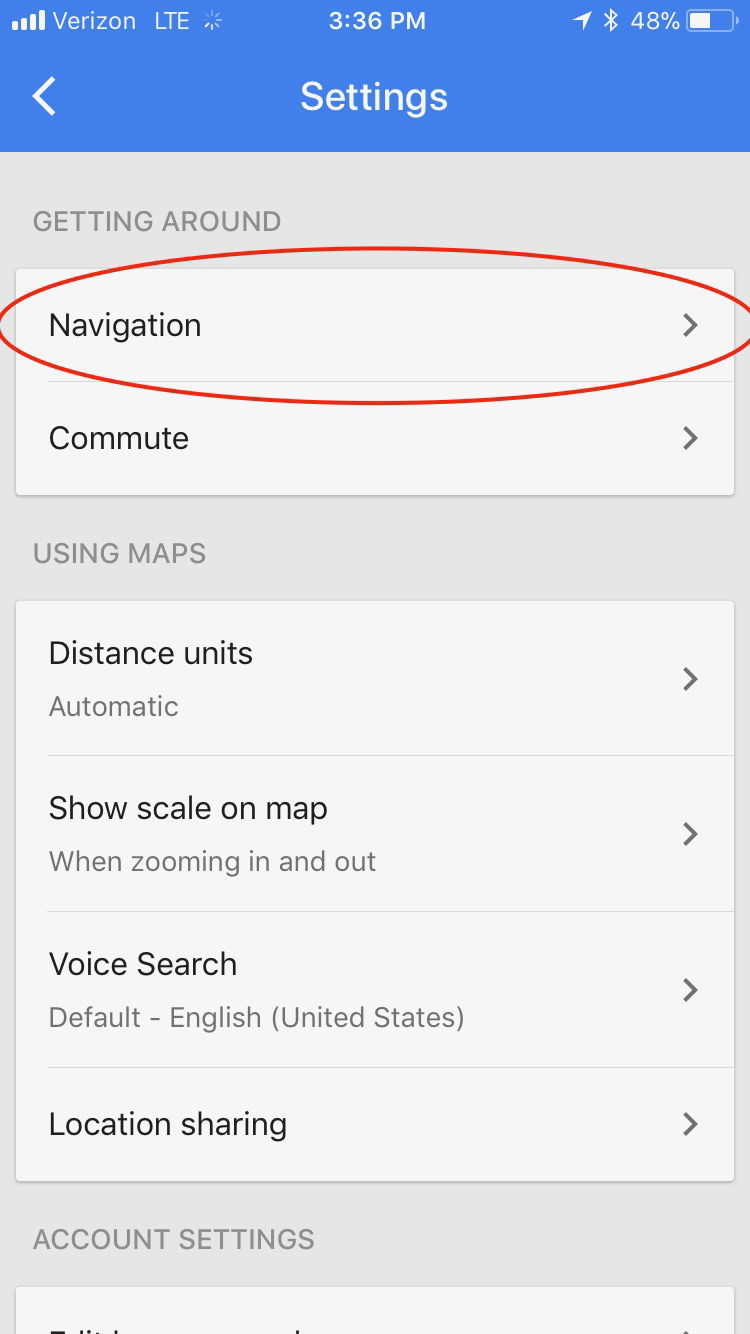This is a detailed screenshot of a phone's settings menu, captured to demonstrate a specific configuration process. The phone, connected to Verizon LTE with a full service signal, displays the time as 3:36 PM. The screenshot also indicates that Bluetooth is enabled and the battery is at 48%.

At the top of the screen, there is a prominent blue box labeled "Settings" with a back arrow for navigation. Below this header, the phone's settings are organized under the category "Getting Around." Within this category, the options "Navigation" and "Commute" are listed, with "Navigation" highlighted by a red circle, likely for tutorial purposes.

Further down, another section labeled "Using Maps" is visible. This section includes the following settings: "Distance units" set to automatic, "Show scale on map" set to display when zooming in and out, "Voice search" set to the default English (United States), and "Location sharing."

At the bottom edge of the screen, another partial header for "Account settings" is visible. The overall interface features a light gray and white color scheme with text in black or dark gray for readability.